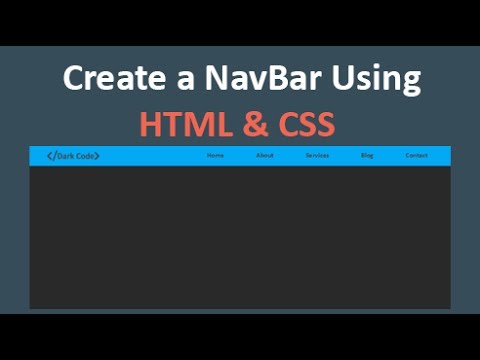This instructional graphic is designed to teach viewers how to create a navigation bar (nav bar) using HTML and CSS. At the top center of the image, there's a title that reads, "Create a Nav Bar Using HTML and CSS." 

Below the title, the graphic showcases a visual example of a navigation bar, dedicated to demonstrating the end result of the coding instructions. The nav bar features a placeholder logo on the left labeled "Dark Code" and five horizontally aligned menu items labeled: Home, About, Services, Blog, and Contact.

The nav bar is styled with a bright blue background, offering a marked contrast against the dark gray background of the rest of the image. This design choice emphasizes the nav bar, making it the focal point of the graphic. The menu items are evenly spaced, contributing to an organized and aesthetically pleasing layout.

The overall design leans towards minimalism, utilizing a sleek black and teal color scheme. This simplistic yet effective design approach ensures that the navigation bar is both functional and visually appealing.